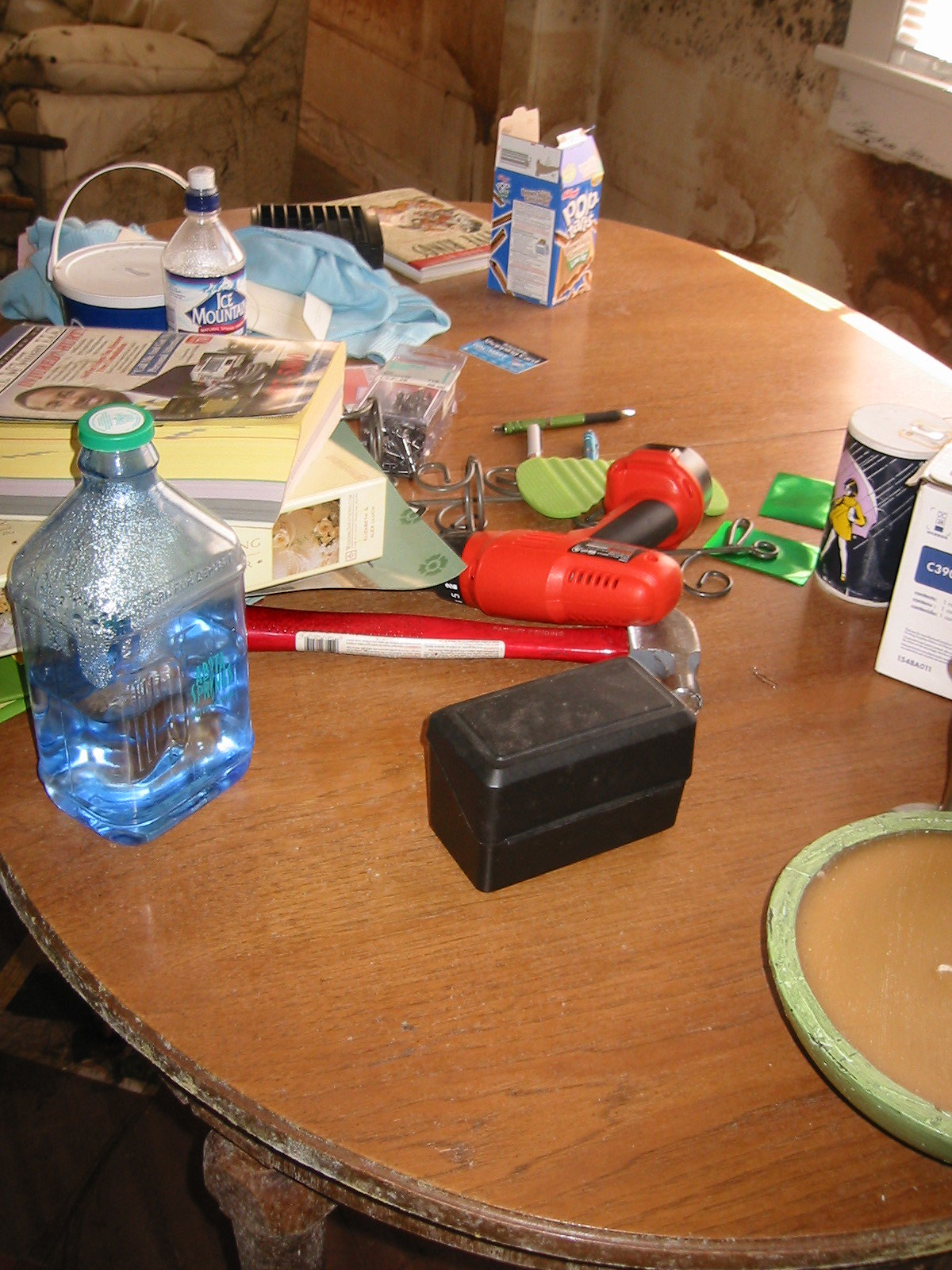The photograph captures a lived-in dining room scene, centering on a slightly worn, brown oval wooden table positioned near a window. Various items are scattered across the table, telling the story of a busy household. In the upper left corner of the image, a reclining chair can be seen, suggesting an adjacent living space. 

On the table, there is a mix of books, though their titles are not discernible. A large juice bottle filled with water stands prominently alongside a smaller bottled water, perhaps Dasani or Ice Mountain. An incongruous bucket is also present, next to a folded blue cloth. The remnants of a meal or snack are evident with an open Pop-Tart box. Tools and household essentials are dispersed among the clutter: an electric screwdriver, a black box, and a small container of Morton's salt, easily identifiable with its green outline. This snapshot offers a glimpse into a moment where everyday life and convenience converge on a well-used dining surface.